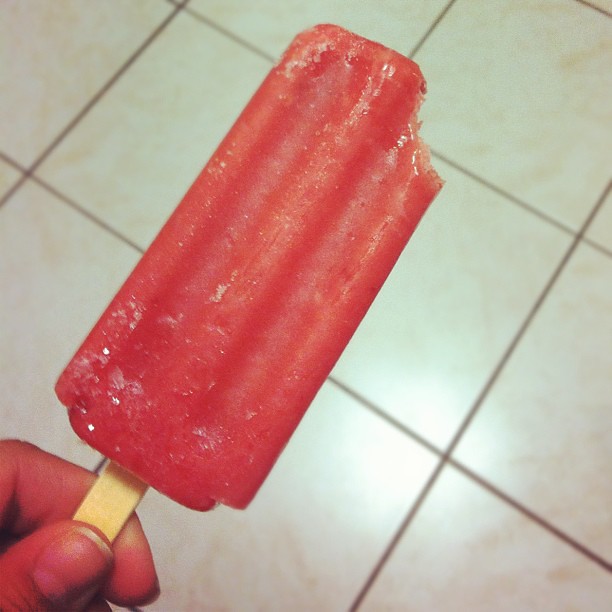This close-up photograph captures a single hand holding a pinkish-red popsicle, with an evident bite mark on its top right corner. The hand, specifically the thumb and index finger, appears in the bottom left corner, pinching the beige wooden stick. Most of the hand is out of the shot. The backdrop is a tiled surface, likely a kitchen floor, featuring beige or cream-colored tiles with brown or gray grout, suggesting a slightly older, possibly blurry photograph. The image does not include any text or date, highlighting solely the interaction between the hand and the partially consumed ice pop.